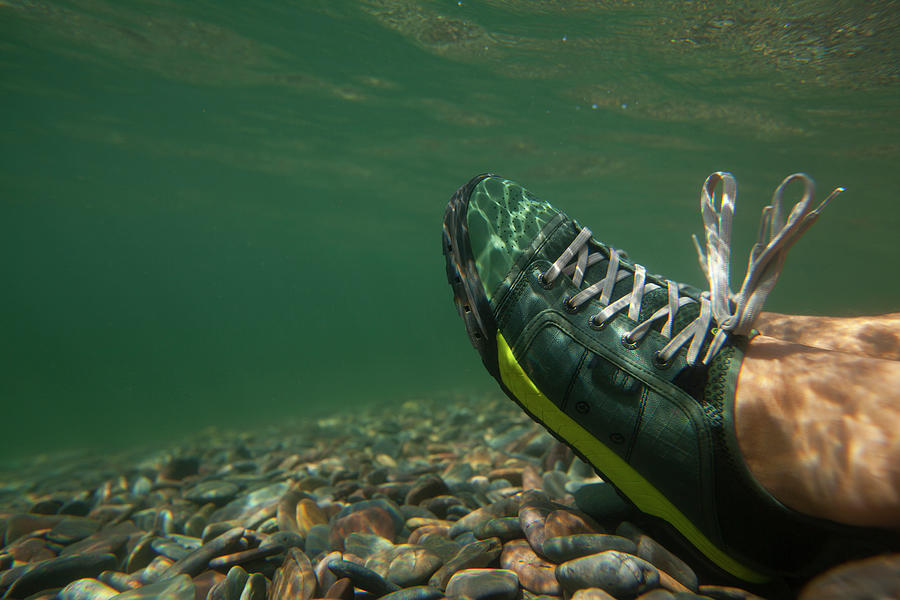This image captures a single green running shoe, detailed with white laces, a lime-green midsole, and a black outer sole, submerged underwater. The shoe rests on a riverbed abundant with small, round, smoothed stones of varying colors, including dark teal blue. The water has a greenish hue, casting reflective patterns on the surface of the shoe. The foot in the shoe is bare at the ankle, extending up to a cropped shin, indicating that the individual is wearing shorts. The shoe is positioned at a diagonal angle, with the heel on the ground and toes angled upward, making it appear almost floating amidst the riverbed scene. The overall vibrant colors and calm underwater setting offer a tranquil and detailed visual.